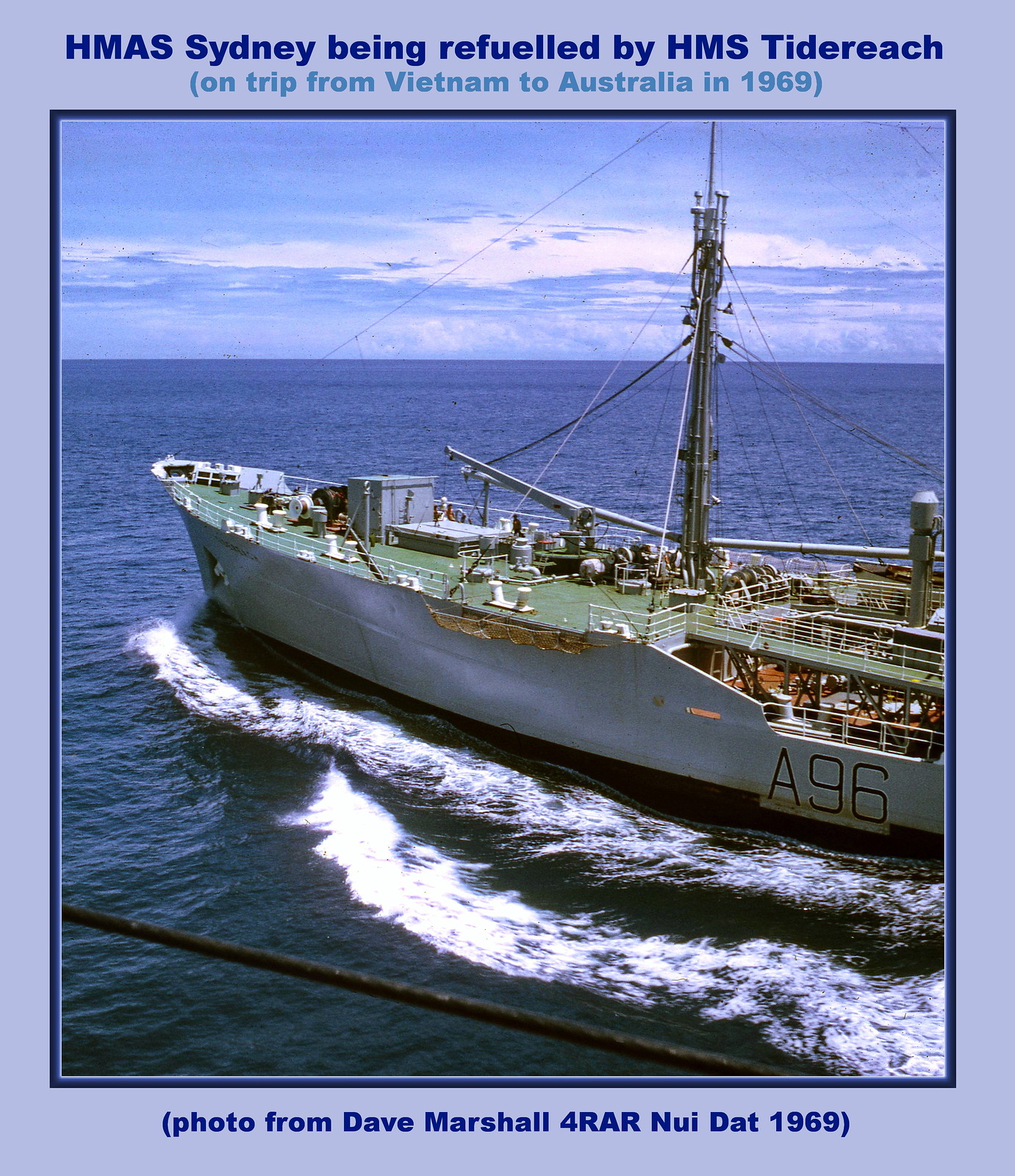This detailed photograph shows a large white and black ship, identified by the markings "A96" on its side, navigating through the open ocean. The backdrop of the scene includes a clear blue sky meeting the horizon, emphasizing the calm yet expansive waters surrounding the vessel. The ship appears to be an army ship, possibly a naval vessel, seen without any sails but exhibiting powerful movement as waves break around its hull. The image appears to be taken from another ship, with visible ship railings framing the foreground.

Above the photograph, blue text reads, "HMAS Sydney being refueled by HMS Tide Reach," and just below that, in a lighter blue, it states, "on trip from Vietnam to Australia in 1969." Below the image, another caption in dark blue text within parentheses states, "photo from Dave Marshall, 4RAR, Nui Dat, 1969."